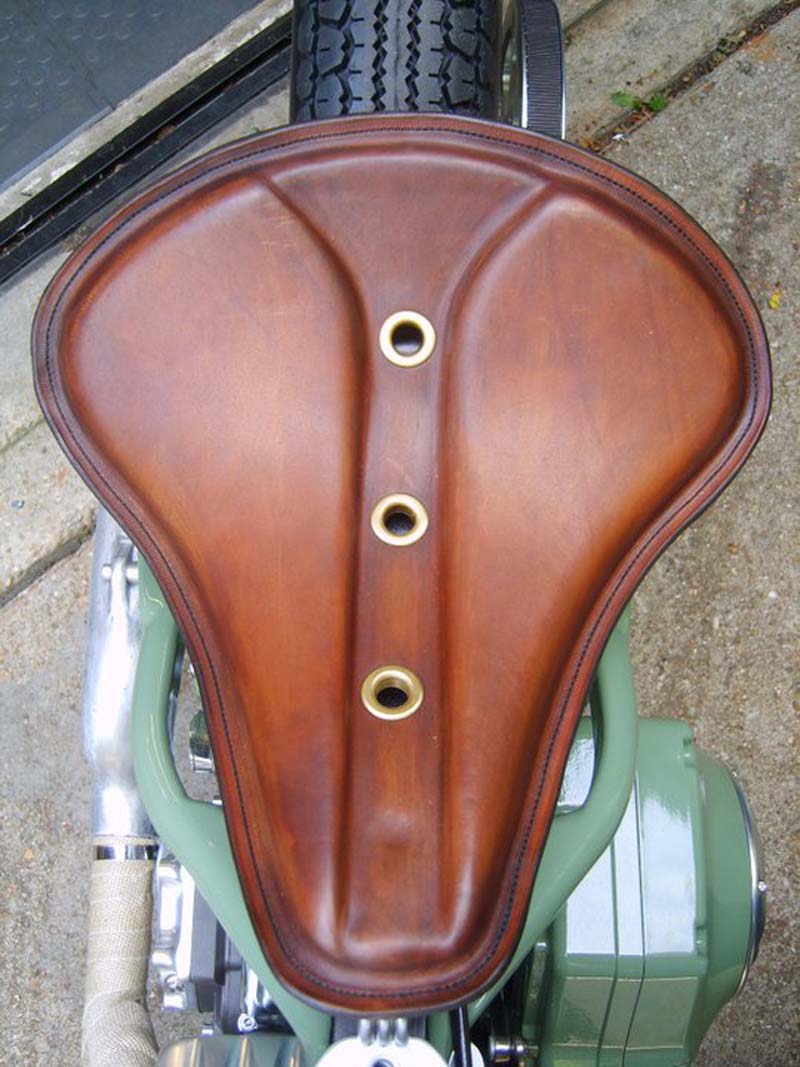This top-down photograph showcases a handcrafted, brown leather seat of a vintage moped or motorcycle, designed in a wide saddle style. The seat is notable for its high-quality craftsmanship and features three gold ring grommets in the center, likely intended for airflow. The grommet holes are set in a depressed channel between two cushioned pads on either side, enhancing the seat's uniqueness and functionality. The moped, shown against a pebbled concrete surface, reveals parts of its beautifully polished, light pastel green frame below the seat. The tire is visible at the top center of the image. On the right side, a component, possibly the carburetor, is seen jutting out, while on the left side, the shiny metallic exhaust pipe is wrapped in a gauze-like tape. The overall impression is one of a well-maintained, classic vehicle with intricate details and a striking, handcrafted appeal.